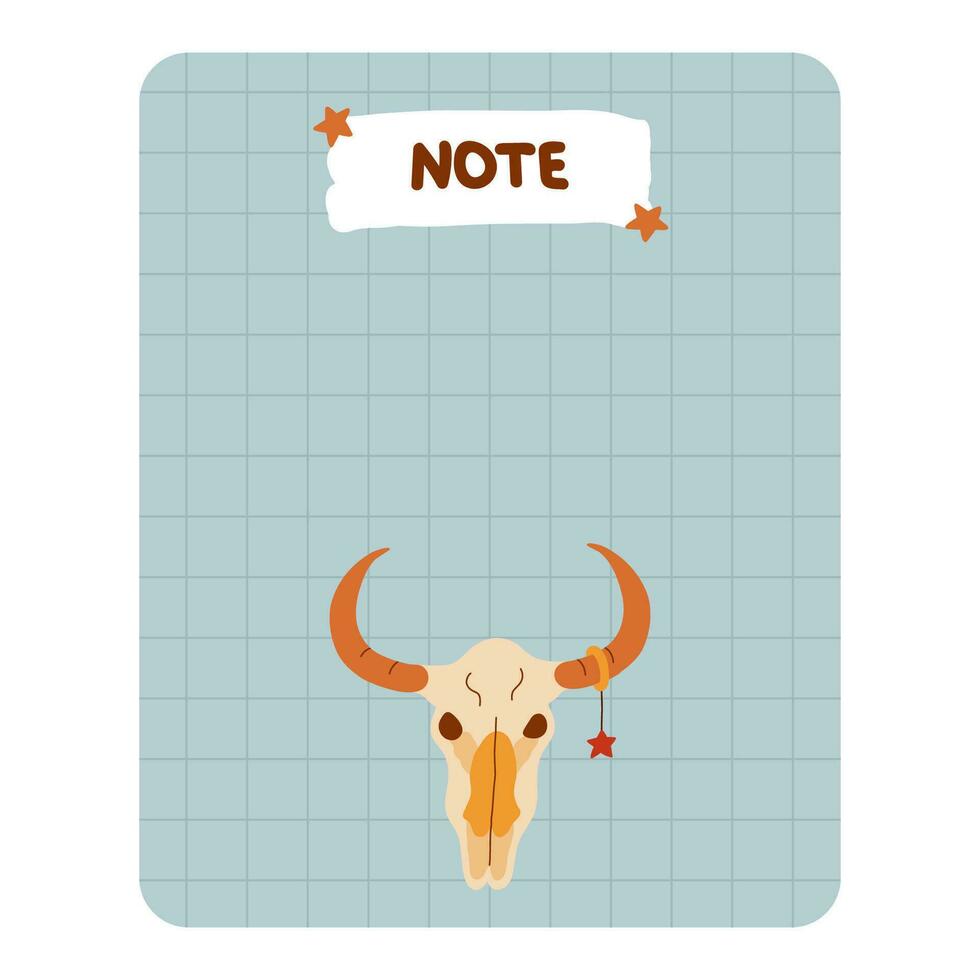This vertical rectangular illustration, likely created with a computer program, features a light turquoise background with a grey grid pattern of evenly spaced horizontal and vertical lines. At the top of the image, there's a white banner offset by two light brown stars, displaying the word "NOTE" in a handwritten style. Below the banner is a detailed clip art image of a buffalo skull reminiscent of those seen in Western movies, complete with pronounced horns and dark brown eye sockets. Attached to one of the horns is a red star hanging from a light brown ring.